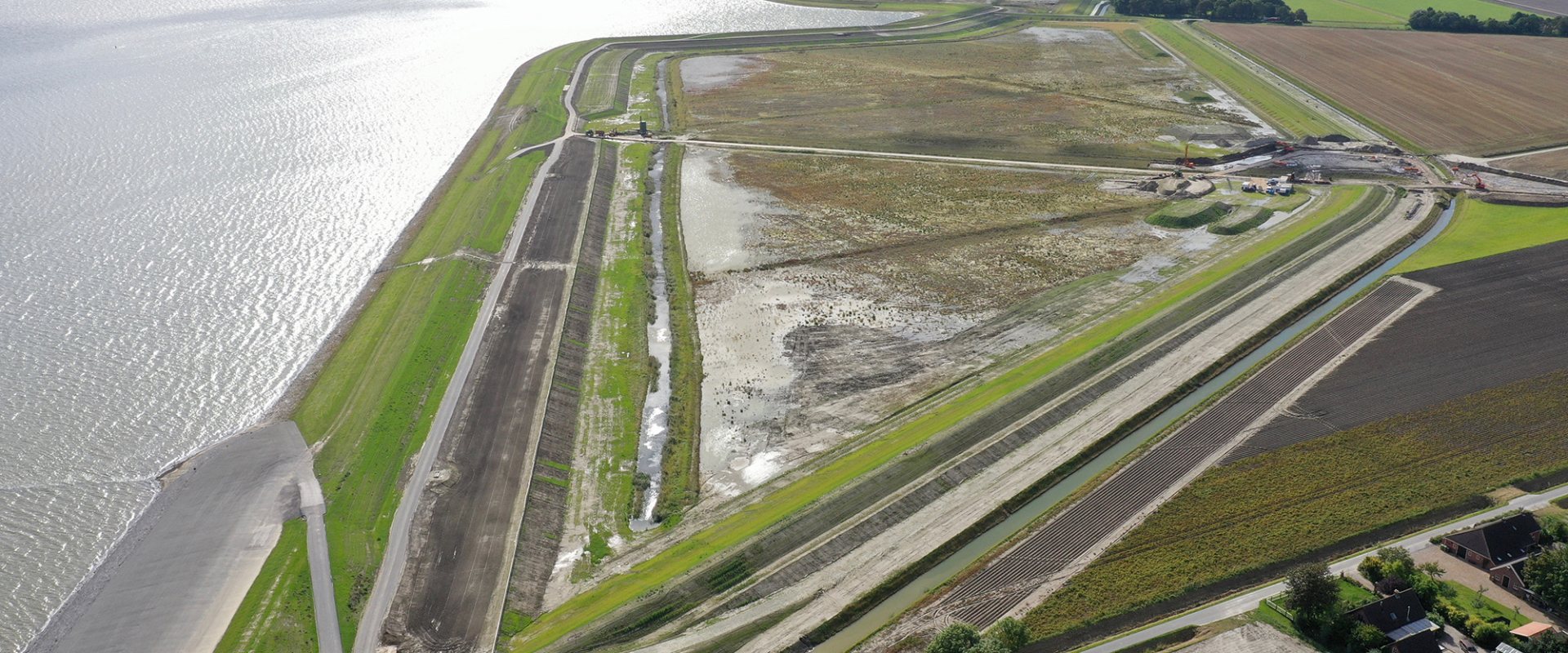This near-horizontal rectangular photograph captures a stretch of well-manicured land, juxtaposed against a serene, grey, and shimmering body of water on the left. The shoreline is graced by a narrow strip of vivid green grass, giving way to a network of transportation paths, possibly asphalt roads, dotting the landscape with precision. These roads weave around large sections of dark brown, well-tended soil that could be areas designated for farming. These sections are intriguingly shaped and seem to be segmented into triangular plots, appearing to be flooded, possibly for crop cultivation. Beyond this, on the right, the farmland continuity is evident with more cultivated fields visible. Despite the agricultural clues, the layout's systematic and interconnected pathways hint at a dual purpose, potentially even that of a small airport, indicating its versatile and accessible nature. The grey sky above, devoid of vibrant hues, adds a calm, overarching ambiance to this meticulously maintained expanse.